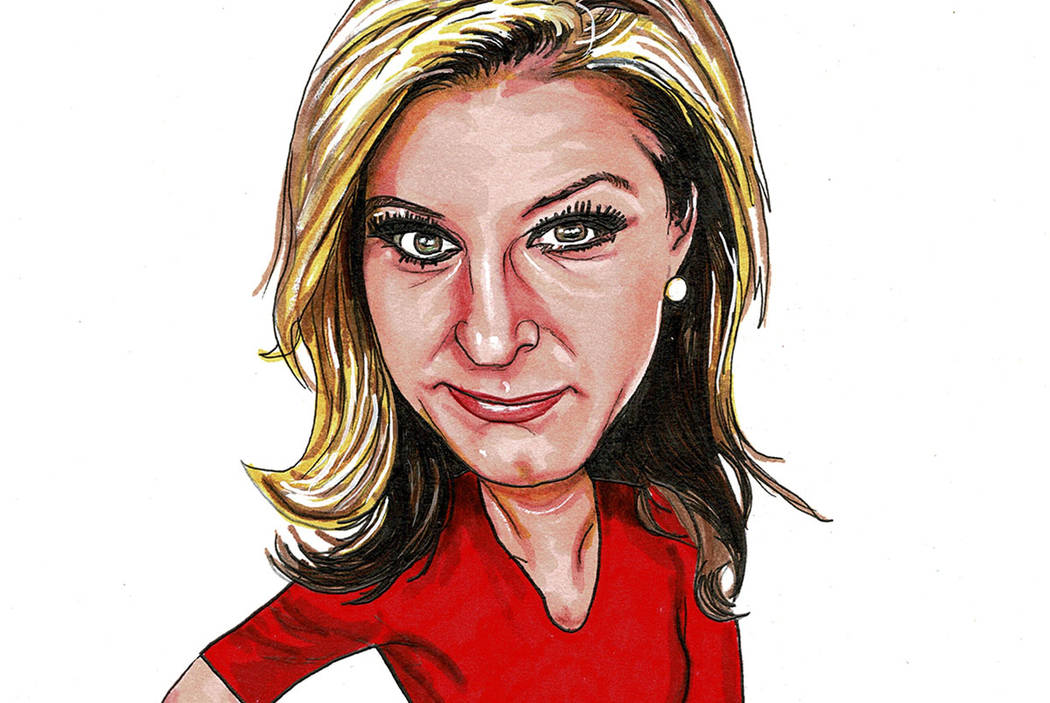This digital drawing features a cartoon-like, close-up portrait of a woman with an exaggerated, disproportionate appearance. Her large head dominates the image, with her body and neck appearing much smaller. The woman has flowing blonde hair, extending to her shoulders with ends that flip outward. She gazes sternly at the viewer with big greenish eyes accentuated by heavy mascara. She wears a pearl-style white earring, visible on one side of her face. Her outfit includes a red V-neck top with three-quarter sleeves, revealing part of her neck and upper arms. The background is entirely white. Details like pronounced shadows add depth, highlighting the creases on her face and enhancing the caricature effect. The color palette is predominantly white, yellow, red, and natural skin tones.